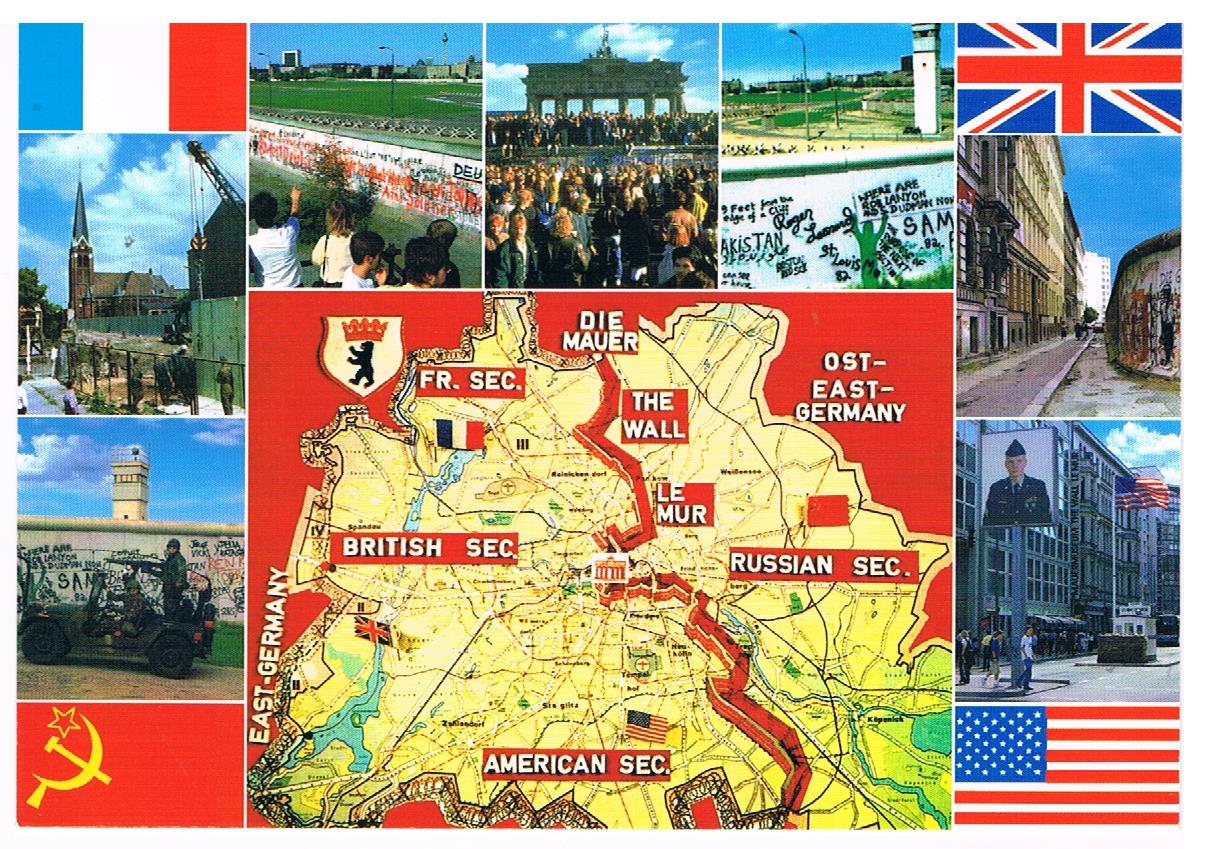The image is a detailed and colorful map of Germany from the era of the Berlin Wall, highlighting the division between East and West Berlin. The map itself prominently features the Berlin Wall, delineated by a red squiggly line running through it. Specific occupational sectors are marked with the flags of the controlling countries: the French sector in the upper left, the British sector on the left, the American sector below that, and the Russian sector to the right, which extends into a larger area labeled as East Germany. The map has a yellow background with a red border. In addition to the central map, there is a collage of pictures surrounding it, showcasing various elements related to the era, such as military presence, significant structures, and public gatherings. These pictures include iconic locations and monuments from the respective countries, contributing to a vivid portrayal of the geopolitical landscape at the time. The flags of France, the UK, the USA, and Russia further decorate the map, emphasizing the division and international influences in Berlin.